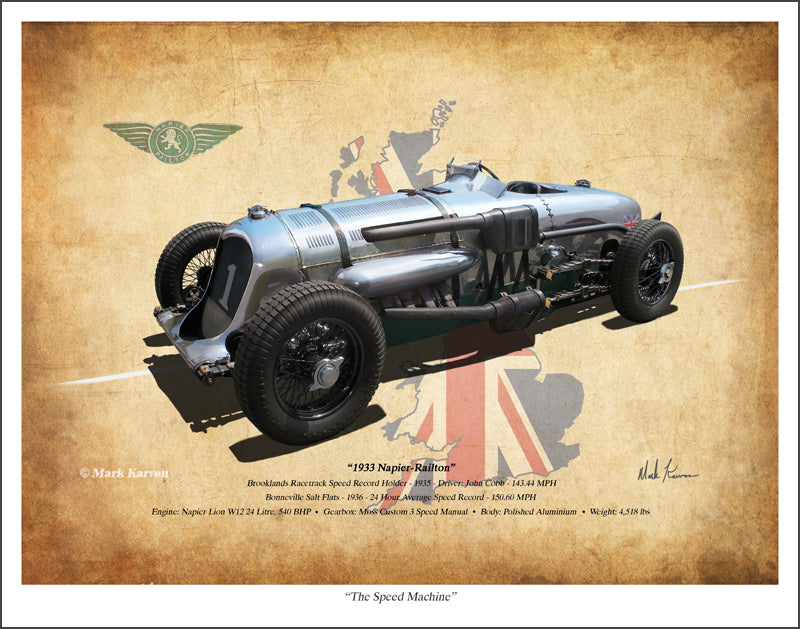The image is a detailed artwork of the 1933 Napier-Railton, prominently displayed as a piece of vintage memorabilia on an old, weathered, brown piece of paper. The paper darkens towards the edges and appears slightly wrinkled, enhancing the nostalgic feel. The centerpiece is the gray, tubular, steel vehicle, which has a distinctive retro look characteristic of the 1920s or 1930s, coupled with unique wheels that lack hubcaps. The car’s design features a small back seat with an exposed steering wheel and visible engine components, adding to its antique charm.

In the background, a map of Great Britain is overlaid with the Union Jack, colored in red, white, and blue, symbolizing the car's British heritage. To the top left, the car's logo, in green and white, is prominently displayed. Beneath the vehicle, text provides historical context: "1933 Napier-Railton, Brooklands’ racetrack speed record holder, 1935," highlighting driver John Cobb and his record speed of 143.44 miles per hour. Additional information mentions a further speed record of 150.6 miles per hour at the Bonneville Salt Flats, along with technical specifications including the vehicle’s weight of 4,518 pounds.

At the very bottom of the image, the car is fondly nicknamed "The Speed Machine," with a signature by the artist, Mark Carman, on the bottom right-hand side, completing this commemorative piece.